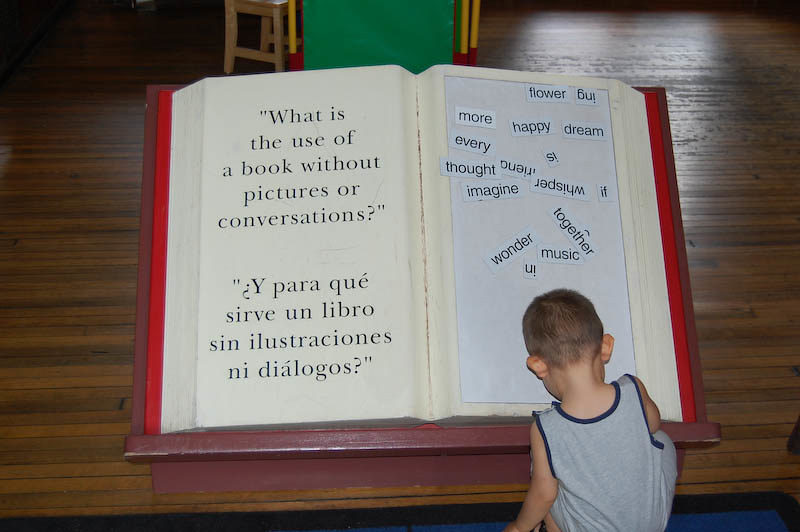The image captures an indoor scene featuring a large wooden sculpture of an open book, prominently displayed on a wooden platform resembling a stage. The book, about the height of a young boy, has text on its left-hand page that reads "What is the use of a book without pictures or conversations?" with a Spanish translation directly beneath it. The right-hand page features an assortment of cut-out magnetic words, allowing for interactive play to form various sentences. Words like "flower," "happy," "dream," and "imagine" are clearly visible, some arranged haphazardly and capable of being repositioned. A young boy, approximately six years old with close-cropped brown hair and wearing a gray tank top with a blue collar, is actively engaging with the display, likely rearranging the magnetic words. The scene is set in what appears to be a children's museum or an amusement area, characterized by additional playful elements like a small chair and a green display in the background. This interactive display provides ample space for children to explore and have fun while sparking their creativity and imagination.